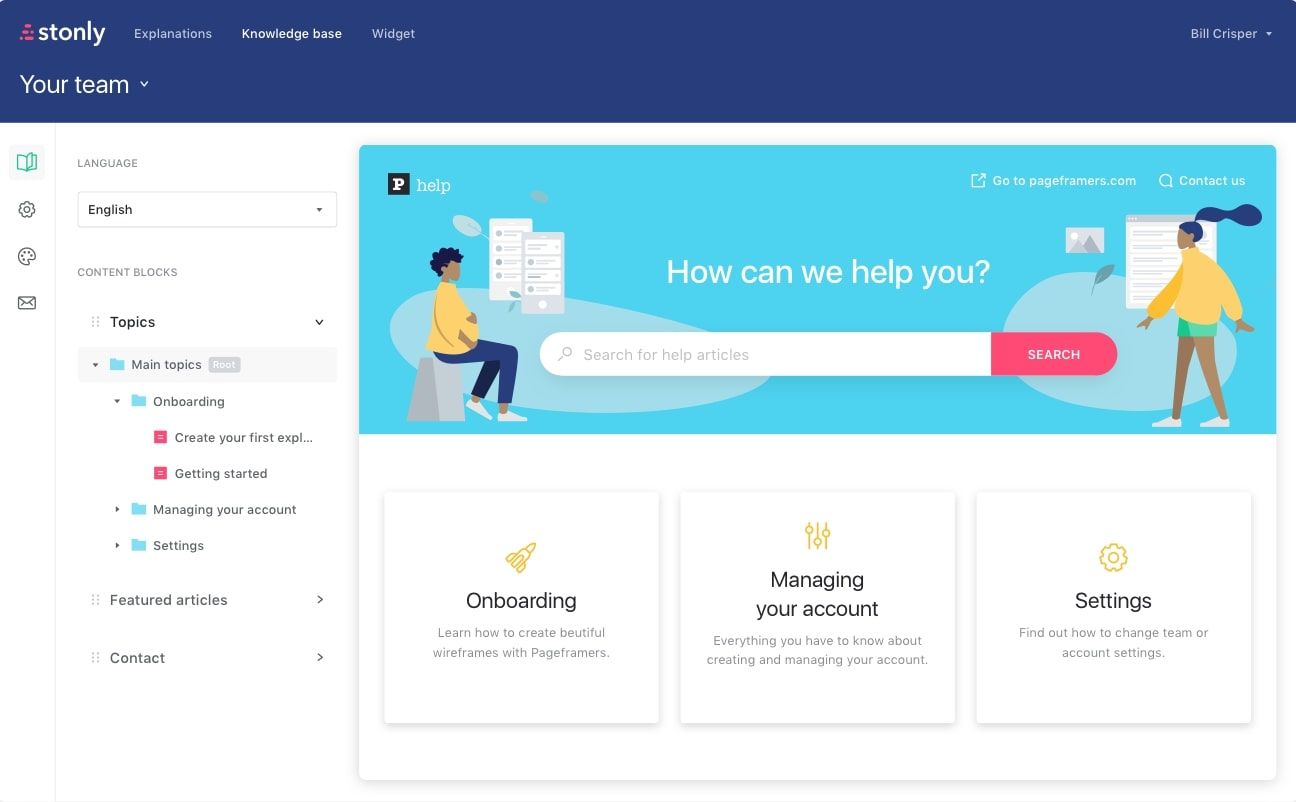### Detailed Image Description:

The image represents a section of the "Stonely" website. The top of the web page features a dark blue header. On the left side of this header, there's an icon depicting a pyramid of red bricks. To the right of the icon is the website name, "Stonely," written in white text, followed by the word "Explanations." The term "Knowledge Base" is highlighted in bold white text, indicating the active section. Further to the right, the word "Widget" appears in regular white text. On the far right end of the header is a drop-down menu with the name "Bill Crisper."

Just below the header, "Stonely" is repeated, accompanied by the text "Your Team" with a drop-down menu next to it. The main content area below this header is predominantly white. On the left-hand side, there is a vertical menu featuring several icons: an open book (green to indicate the current selection), settings gear, a paint palette, and an envelope. These icons are separated by a vertical gray line.

Near the top left of the main content area, the word "Language" is displayed in gray text, followed by a drop-down menu that shows "English" in bold, active black text. Below this, "CONTENT BOX" is written in gray capital letters. Alongside, the word "Topics" appears in bold with a drop-down menu next to it. Under this section, there is a blue file folder icon labeled "Main Topics," accompanied by a gray box labeled "Root," which is highlighted.

Further below, another blue file folder icon with a down arrow next to it is labeled "Onboarding." Below this, a red square icon with white lines contains the text "Create Your First Expla..." (ellipsis indicating truncated text). There are additional red and blue boxes labeled "Getting Started," "Managing Your Account," and "Settings," each with corresponding icons and arrows to their left.

On the larger central portion of the webpage, a light blue background dominates. At the top left of this section, a black square with a white capital "P" and the word "Help" in white text are displayed. On the right-hand side, the text "Go to PageFramers.com" and "contact us" are outlined.

Within the light blue section, there's an illustration featuring two overlapping cell phones and a satellite. A black girl with short hair, wearing a yellow shirt and blue jeans, is sitting on what appears to be a rock. The text "How can we help you?" is prominently displayed in large white letters. Below this text is a search bar with the placeholder "Search for help articles." A red area to the right contains the word "Search" in white text.

To the right of this section, there's another illustration of a black girl with a long ponytail, wearing a yellow shirt, green shorts, and white sneakers. Nearby, there's an image of the sun rising over two mountains, with a leaf protruding from a light blue oval background.

Below the blue section, three white boxes are aligned horizontally:
1. The left box has a golden spaceship icon and the header "Onboarding" in black text. It provides information on creating beautiful wireframes with Page Framers.
2. The middle box is related to "Managing Your Account" and contains a vertical slider symbol. It provides details on account creation and management.
3. The right box, with a gold gear icon, is labeled "Settings." It offers information on changing team or account settings.

This comprehensive description details the layered website layout and various interactive elements present on the page.